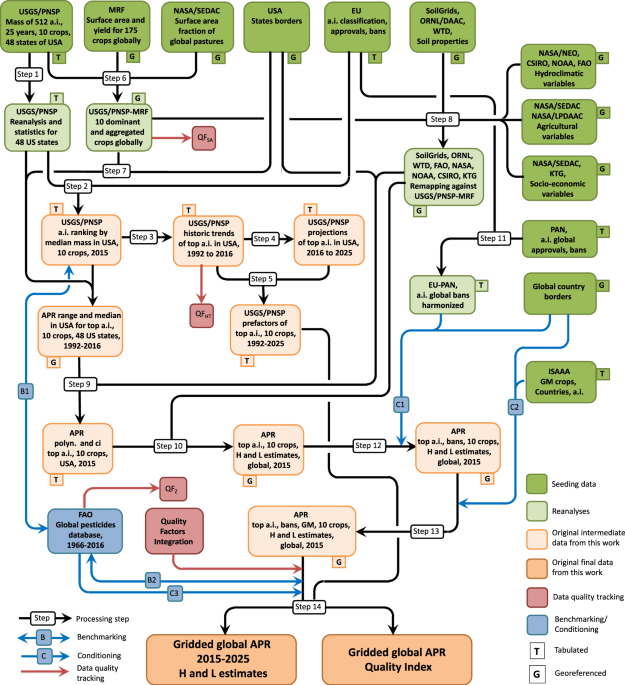The image depicts a complex diagram with various colored rectangles and rounded-edge bubbles interconnected by multicolored lines, including blue, black, and red. The rectangles contain numerous text summaries alongside acronyms and codes such as USGS PNSP NASA 512 AI, covering topics like 25 years of data on 10 crops spanning 48 states of the USA. Additionally, the diagram includes references to MRF and NASA/CDAP surface areas, and various global datasets related to crop yields, pastures, soil properties, and hydroclimatic variables from sources like NOAA and FAO.

Among the boxes, some are solid green, blue, or red, each color representing different types of data stages or categories, like seeding data and benchmarking/conditioning as indicated by a color legend. Bubbles are labeled with terms such as EUPAN, Global Country Borders, Socioeconomic Variables, and Global Approvals.

The bubbles are sequentially connected by arrows that delineate the flow or steps of data processes or classifications. At the bottom of the diagram is a detailed key explaining the different data types including original, intermediate, and final data, along with data quality tracking. The entire chart appears to relate to agronomic and geographic data visualization, likely explaining intricate layers of agricultural analysis or policies.